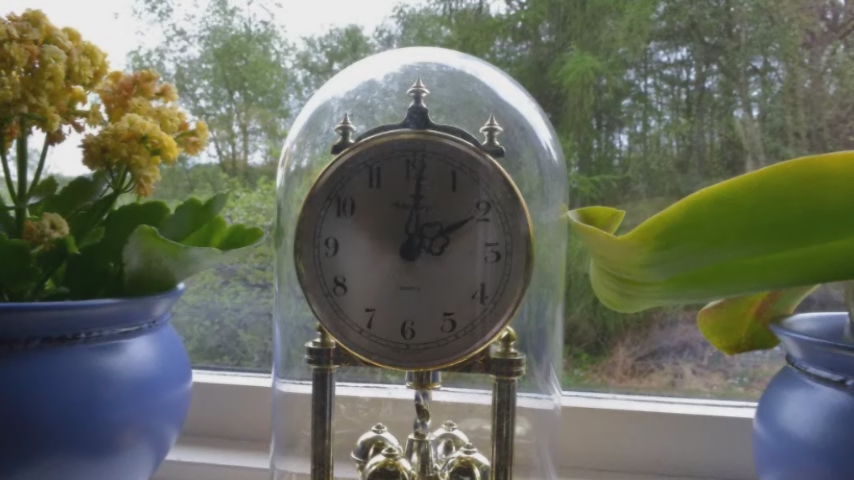Through the window, a serene landscape unfolds, featuring a road winding through gentle rolling hills covered in a lush expanse of trees under a light, pleasant sky. In the foreground, a medium blue flower pot immediately draws attention, adorned with clusters of vibrant yellow flowers and generous green leaves. Beside it, a golden clock commands presence, encased in a clear glass dome, with its black numbers and hands clearly visible against the crisp background. Another blue flower pot complements the scene, showcasing a prominent green leaf that elegantly curls at the tip, with another leaf gracefully draping downward. This charming vignette combines elements of nature and classic design, framed perfectly by the window to create a captivating view.